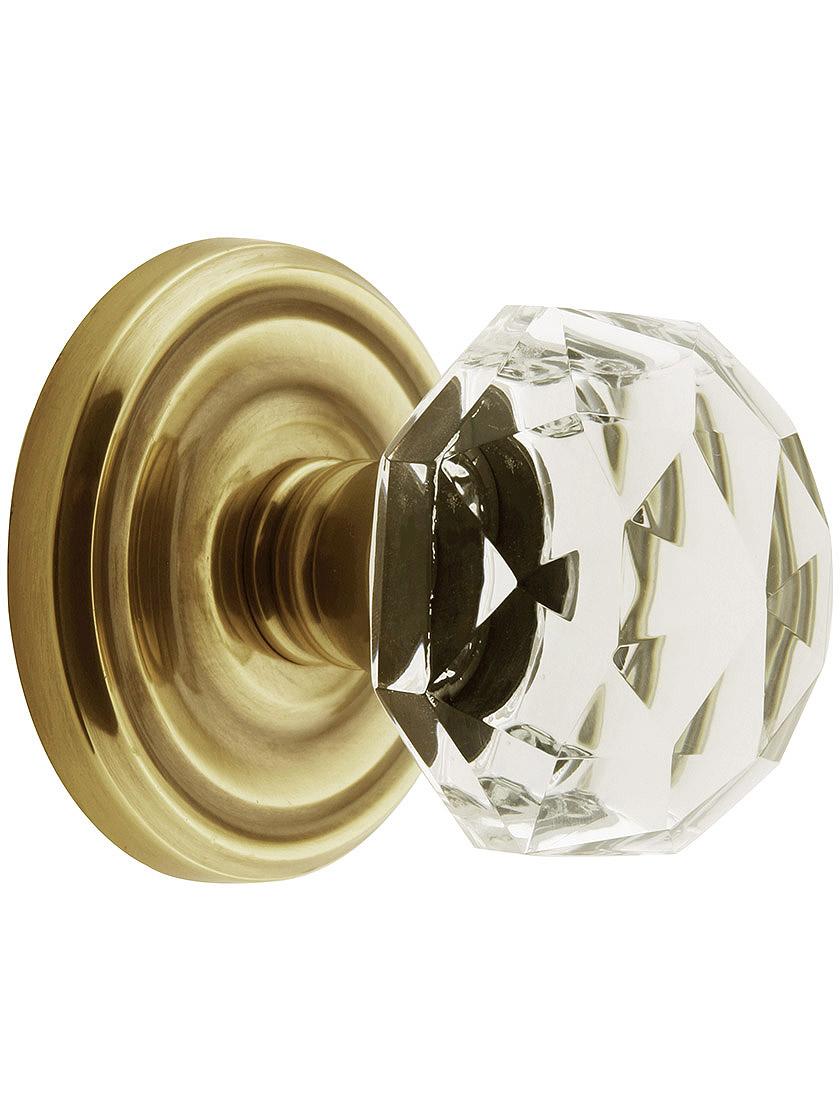This photograph showcases a luxurious doorknob set against a white background in a portrait orientation, emphasizing the opulence of its design. The doorknob features an elegant glass handle designed with a multifaceted, diamond-like pattern, creating a dazzling effect with its numerous curves and edges. This glass component exudes a sense of depth and dimension, sparkling brilliantly and suggesting a high-end, luxury feel. The mounting plate of the doorknob is crafted from circular, brass or gold-toned metal, intricately detailed with ridges and round circles that reinforce the overall sophisticated aesthetic. The pristine condition of the doorknob and its ornate detailing imply that it is a modern reproduction of a vintage style, ideal for upscale homes or opulent settings such as luxury hotels. The doorknob’s weight and the quality of materials used further accentuate its intended market for affluent consumers seeking to enhance their living spaces with tasteful, high-quality fixtures.